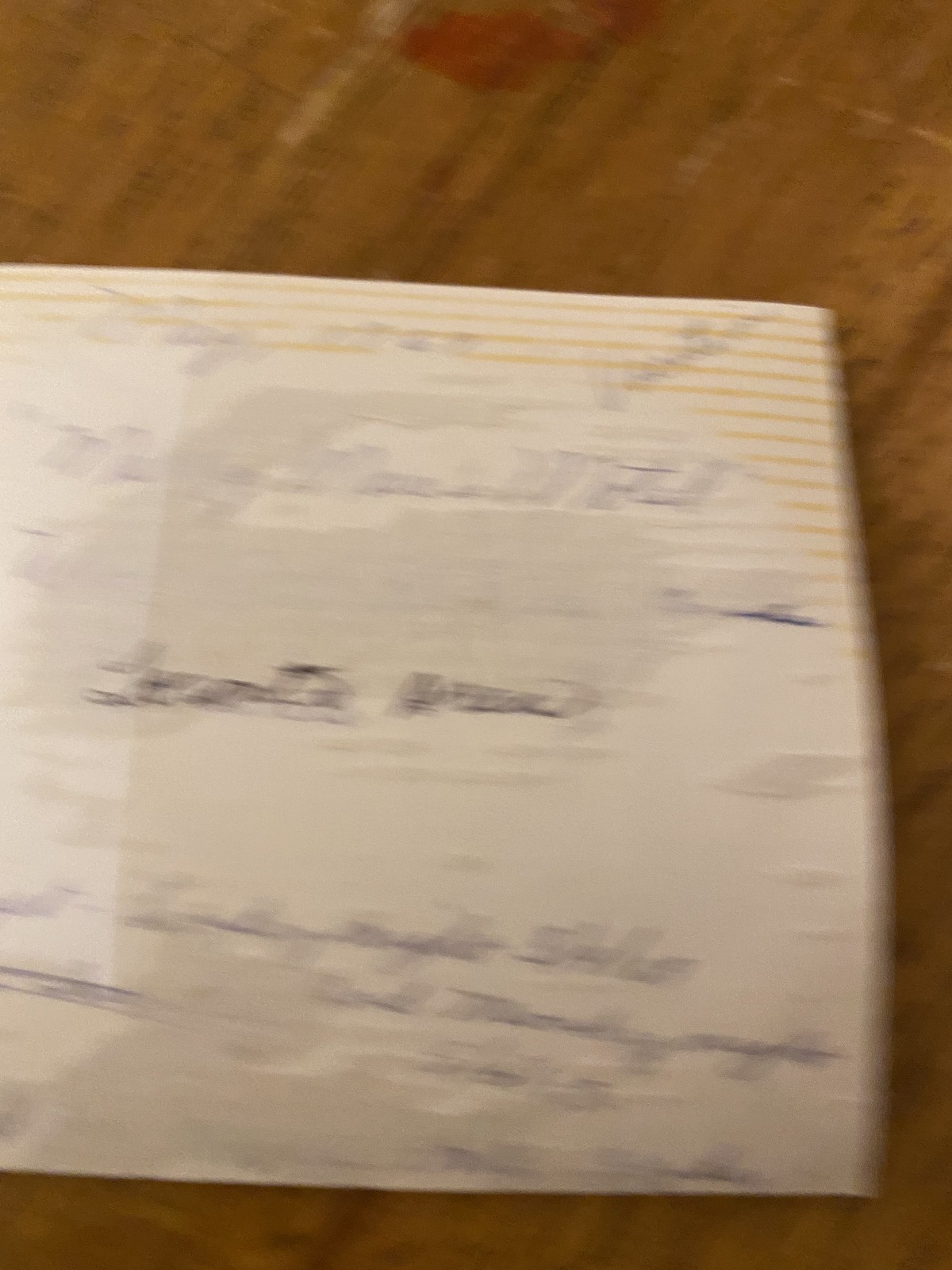This image is a very blurry color photograph that captures a tall, rectangular piece of lined paper set against a brown wooden backdrop. The paper is covered in various styles of handwriting, creating a visually busy but ultimately illegible array of text. The surrounding area, free from any other objects, animals, or people, allows the viewer to focus solely on the indistinct writing. Due to the extreme blurriness, the contents of the written text cannot be discerned, adding a layer of mystery to the overall composition. The photograph's vertical orientation emphasizes the elongated shape of the paper and the wooden texture of the background.